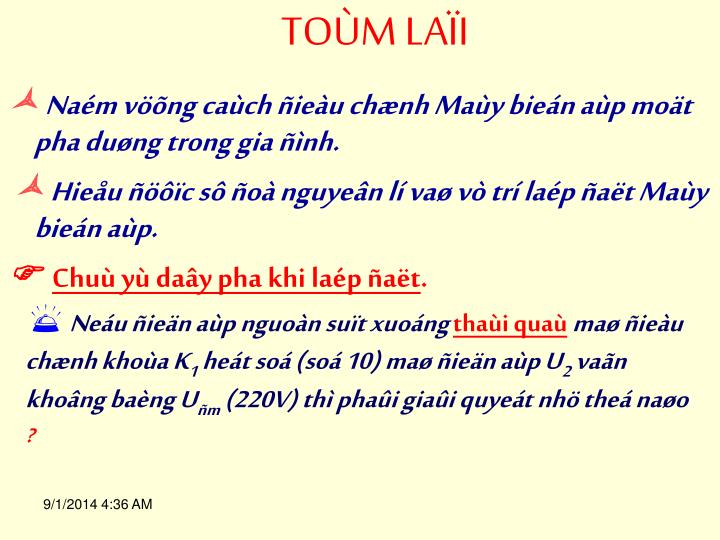The image depicts a PowerPoint slide with a creamy, yellowish-tan background and text in red and blue, written in a foreign language, possibly Indonesian or Vietnamese. At the top center is the title in red, "T-O-U-M L-A-I-I," with distinct accents over some letters. There are three bullet points on the slide: the first two use red three-sided star icons alongside two lines of blue text each. Below these, there is red underlined text next to a pointing finger icon, emphasizing its importance. Further down, a blue service bell icon precedes another line of blue text containing two red and underlined words, along with a red question mark on the fourth line. The slide is timestamped in the bottom left corner with the date 9-1-2014 at 4:36 AM.